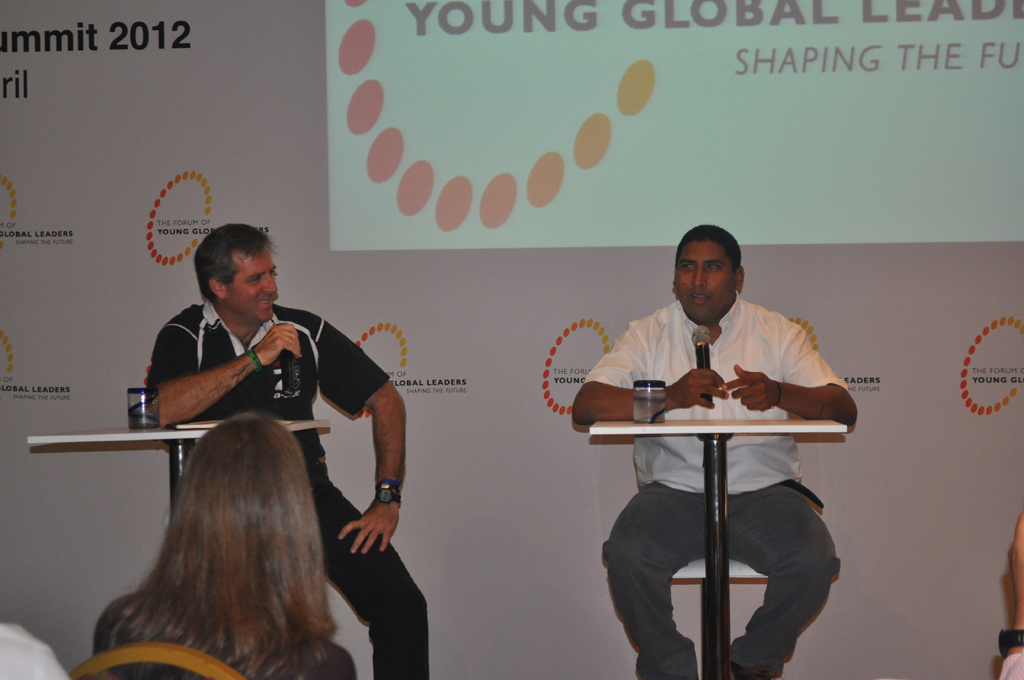The image captures a vibrant scene at a convention or seminar titled "Young Global Leaders Shaping the Future." Prominently displayed on a blue banner with red and orange dots, the title of the event sets the tone. Two male speakers sit at individual small white tables, both equipped with microphones and identical water cups.

The speaker on the left wears a black shirt, black pants, and a wristwatch. He gazes attentively towards his counterpart while holding his microphone. The speaker on the right is clad in a white half-sleeve shirt and grey pants, holding his microphone in his right hand and engaging with the audience. Both tables have similar glass jars.

In the audience, a woman with shoulder-length red hair attentively listens while seated on a yellow chair. The venue is decorated with a repeating logo of red and orange dots, and a projection of a laptop screen displays a partially visible logo and slogan. Additionally, scattered hands in the audience suggest an engaged participation, even though they are not fully identifiable.